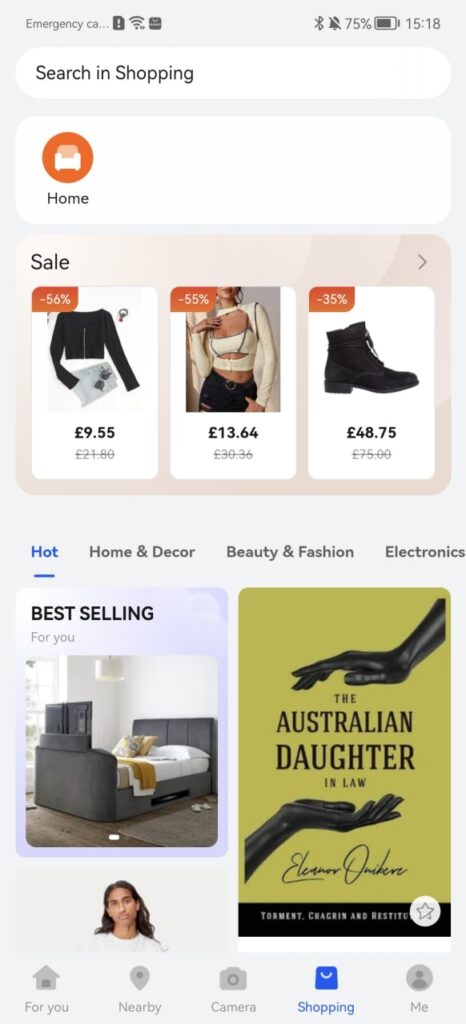The image is a screenshot of an iPhone displaying a shopping app with a light background. At the top, there is a search bar labeled "Search and shopping." Below the search bar is a white navigation bar featuring an orange circular icon with a white house symbol inside it, accompanied by the label "Home."

Directly beneath this navigation bar is a section with a light brown background labeled "Sale" in black text. This section showcases three articles of clothing side by side. 

- The first item is a women's top with a zipper, exposing the midriff, priced at £9.55.
- The second item is another women's top with long sleeves that reveals significant cleavage and some midriff, priced at £13.64.
- The third item is a pair of black boots, priced at £48.75.

Each product has an orange label in the upper left corner of its image, indicating the percentage discount applied to the original price.